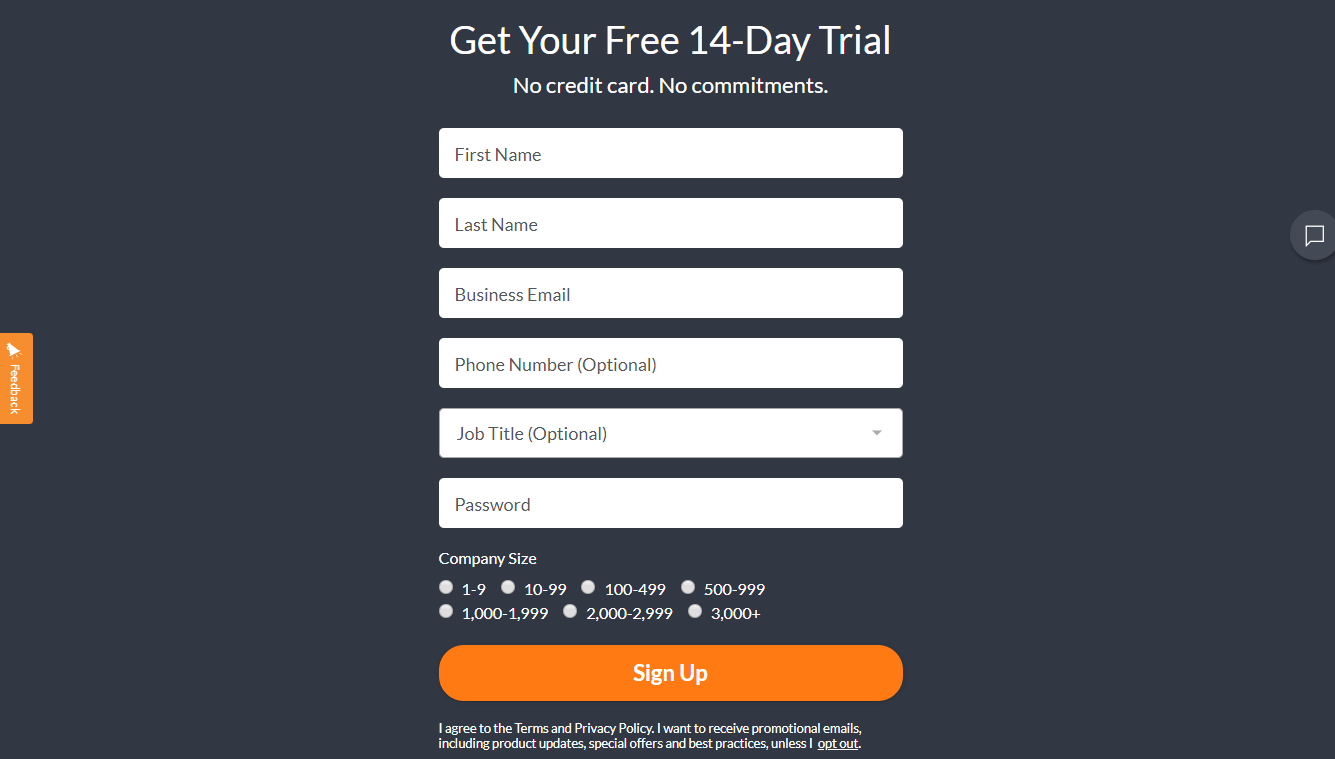The image is a colorful advertisement and signup form, framed to fit a computer screen. It prominently features the text "Get your free 14-day trial, no credit card, no commitments" on a sleek, black background. Below this message is a crisply designed form with white text fields where users can input their:

- First Name
- Last Name
- Business Email
- Phone Number (optional)
- Job Title (optional)
- Password

Additionally, there's a drop-down menu to select the company size with options ranging from "1 to 9" to "3,000+".

At the bottom of the form, there's a large orange "Sign Up" button in white text. Beneath this button, small print states, "I agree to the terms and privacy policy. I want to receive promotional emails including product updates, special offers, and best practices unless I opt out." The phrase "opt out" is underlined, indicating it is a clickable link to opt out of receiving promotional emails while still submitting the form.